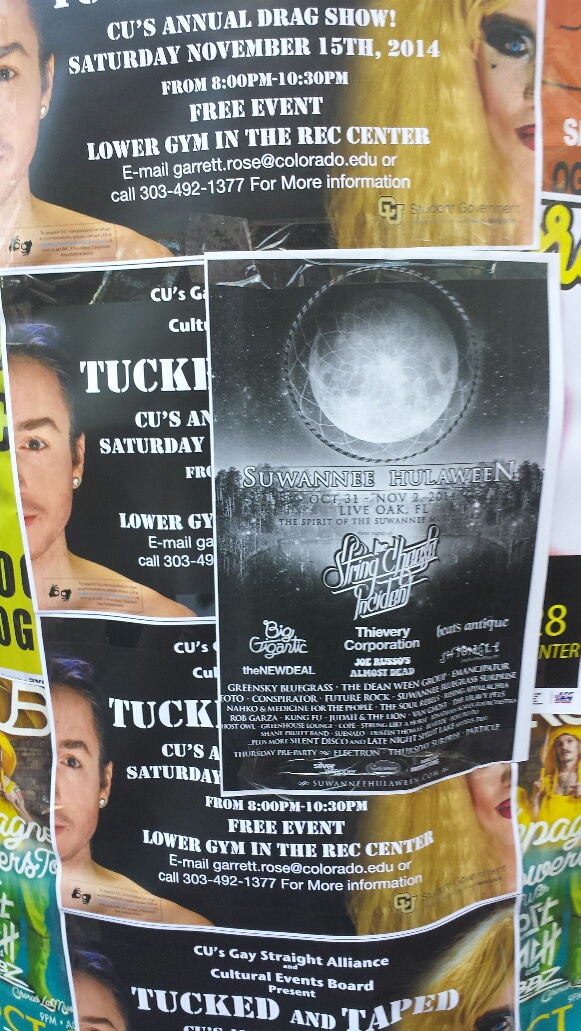The image depicts a series of identical flyers adhered to what appears to be a telephone pole or a streetlamp. These flyers advertise CU's annual drag show scheduled for Saturday, November 15th, 2014, from 8 p.m. to 10:30 p.m. at the Lower Gym in the Rec Center. The flyers are in white lettering and include contact information for Garrett Rose (email: Garrett.Rose@colorado.edu, phone: 303-492-1377). The right side of the flyer features a man in makeup with long blonde hair, while only half of a man's face is visible on the left. All the flyers are arranged vertically, with at least four of them in a row. Overlapping two of the drag show flyers, there is a black and white ad for "Suwannee Hulaween Spring Break Incident," which appears to promote a Halloween-themed event featuring a variety of bands.